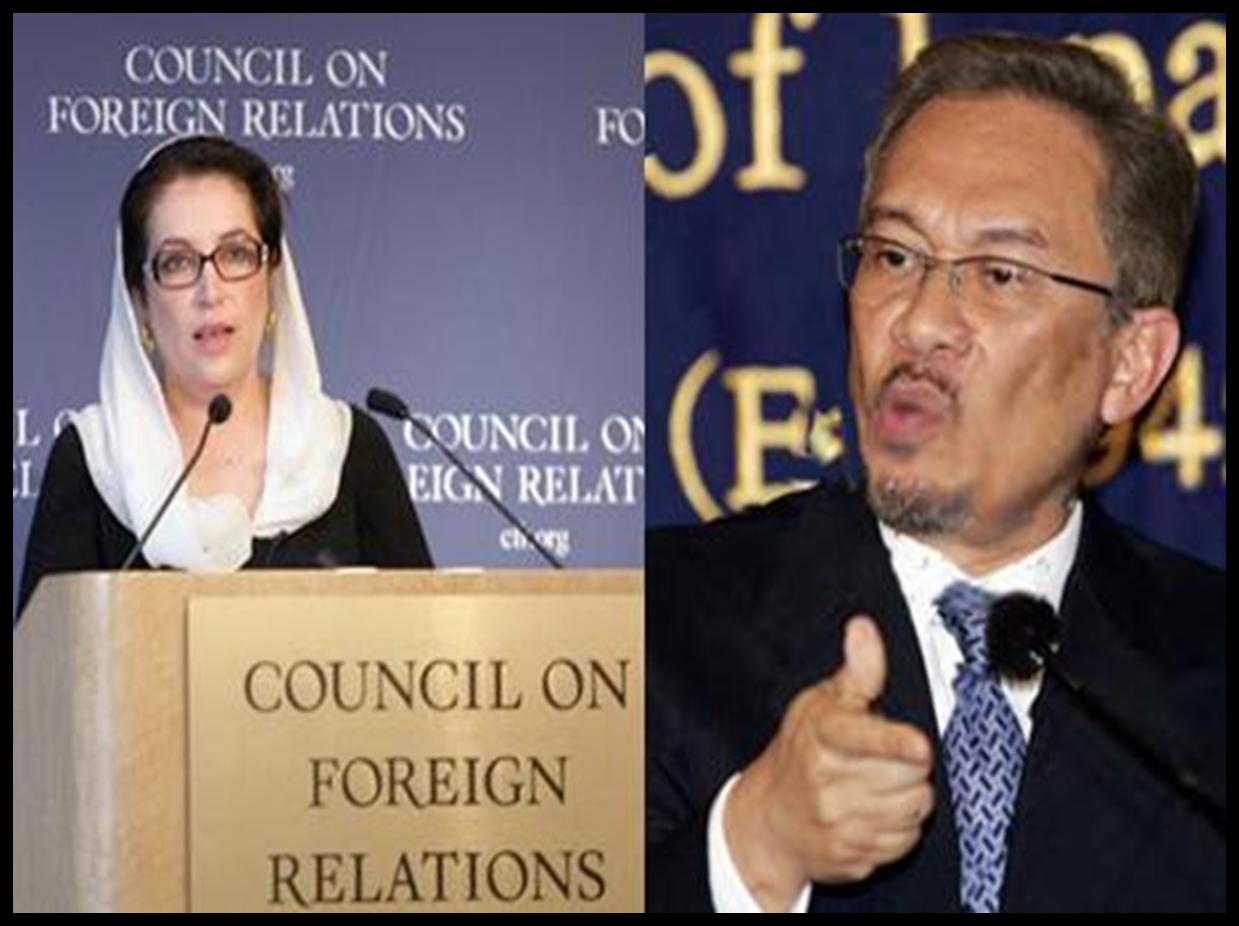The image is a collage consisting of two juxtaposed photographs, formatted in a landscape orientation with a black rectangular border. The left side dominates slightly more space, featuring a woman at a podium. She is adorned in a white headscarf overlaying a black dress or shirt and is captured mid-speech. Her podium bears the inscription "Council on Foreign Relations" in dark text on a brown backdrop, and two baby microphones are positioned toward her face. The backdrop behind her is purple and repetitively emblazoned with "Council on Foreign Relations" in white text.

The right side of the collage presents a man shown from the chest upwards, dressed in a black suit, a white shirt, and a purple tie with black specks. He too appears to be speaking, with his mouth forming an 'O' shape, and gesturing with his right hand. The man, middle-aged with glasses, a small mustache, and a beard, is set against a backdrop the details of which are largely obscured, save for the partially visible word "of." The tight framing makes it difficult to identify the full context or specific background text for him.